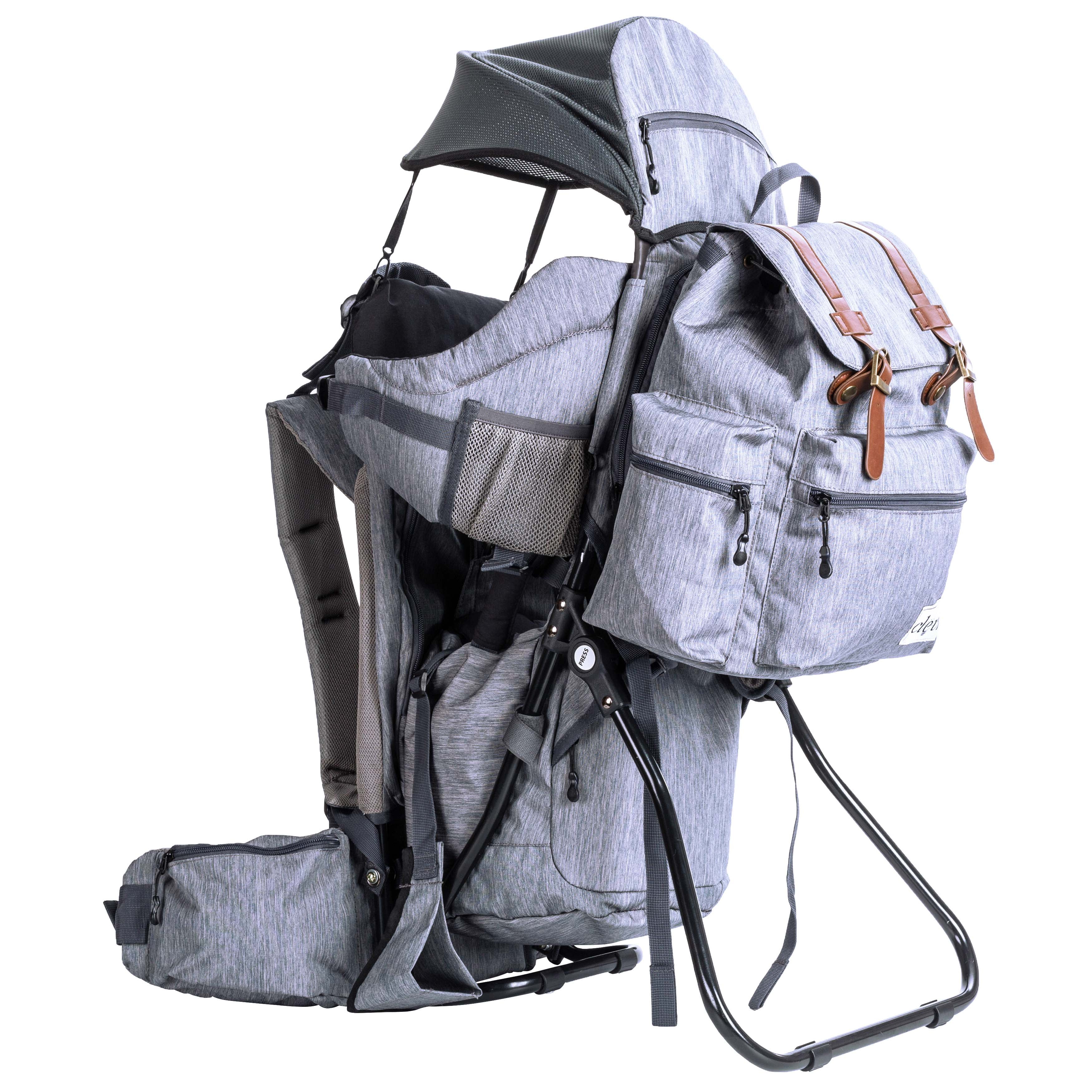This image appears to be a detailed product photograph of a multi-functional backpack designed for outdoor activities, such as camping. The backpack, predominantly in various shades of gray, features a complex structure with multiple attachments and storage compartments. The central element is a large backpack attached to a sturdy black metal frame that includes an upper canopy for weather protection. The fabric is a nuanced gray, resembling a pencil sketch with varying shades, and is complemented by black zippers and pulls. There are several storage areas, including a small pocket and a compartment on the bottom, as well as a concealed, foldable chair-like seat, possibly intended for carrying a small child. Additionally, a secondary smaller backpack with brown leather straps and a front pocket is attached to the main structure. The entire setup, depicted against a white background, suggests a versatile and robust design ideal for extended outdoor use.